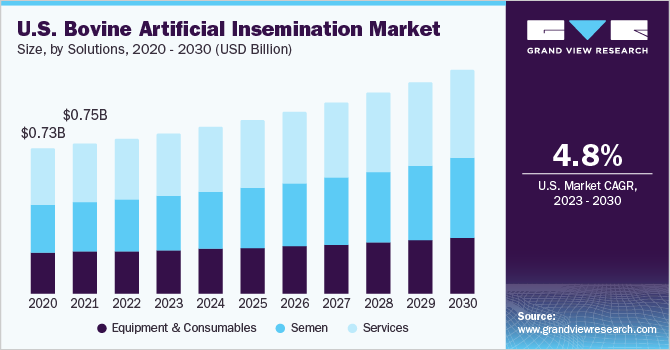This image is an infographic slide featuring a bar chart titled "U.S. Bovine Artificial Insemination Market Size by Solutions 2020-2030 (USD Billion)." According to Grandview Research, the market has a compound annual growth rate (CAGR) of 4.8% from 2023 to 2030. The chart, sourced from www.grandviewresearch.com, displays annual market size starting at $0.73 billion in 2020 and $0.75 billion in 2021, with a continuous upward trend until 2030. The bars are color-coded: purple represents equipment and consumables, blue indicates semen, and light blue signifies services.